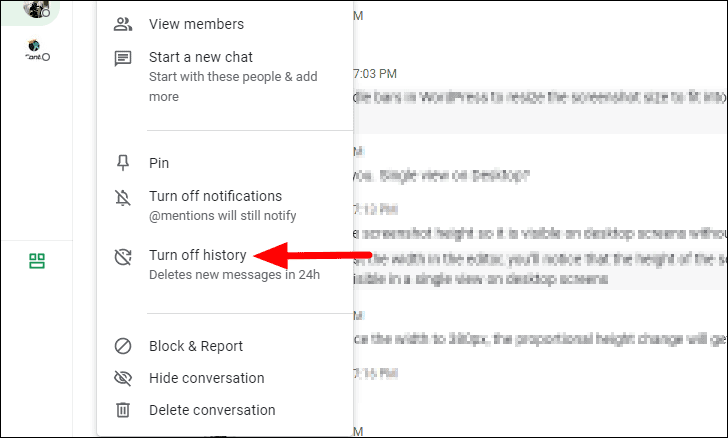The image is a screenshot from a website, framed by a thin black border. On the left side of the image, there is a spanner icon that is partially cut off at the top. Near this icon, there's a small graphic with some text, but part of it is also cut off, making it partially unreadable. 

Prominently featured in the image is a white pop-up menu. Running down the side of this menu are several small icons. Next to these icons are text options. The first option is "View Members," starting with a capital "V." Below that, the next option reads "Start a New Chat," with a subtitle that says, "Start with these people and add more." 

A dividing line separates these options from the next set. The subsequent options listed are "Pin," "Turn Off Notifications" (with a note indicating that mentions will still notify), and "Turn Off History." A red arrow from the side points to the "Turn Off History" option. Underneath this, another option reads, "Delete New Messages in 24 Hours."

Further down, there is another small dividing line, after which the following options are listed: "Block and Report," "Hide Conversation," and "Delete Conversation."

The pop-up menu obscures some underlying text on the webpage, which appears distorted and unreadable due to digital artifacts.